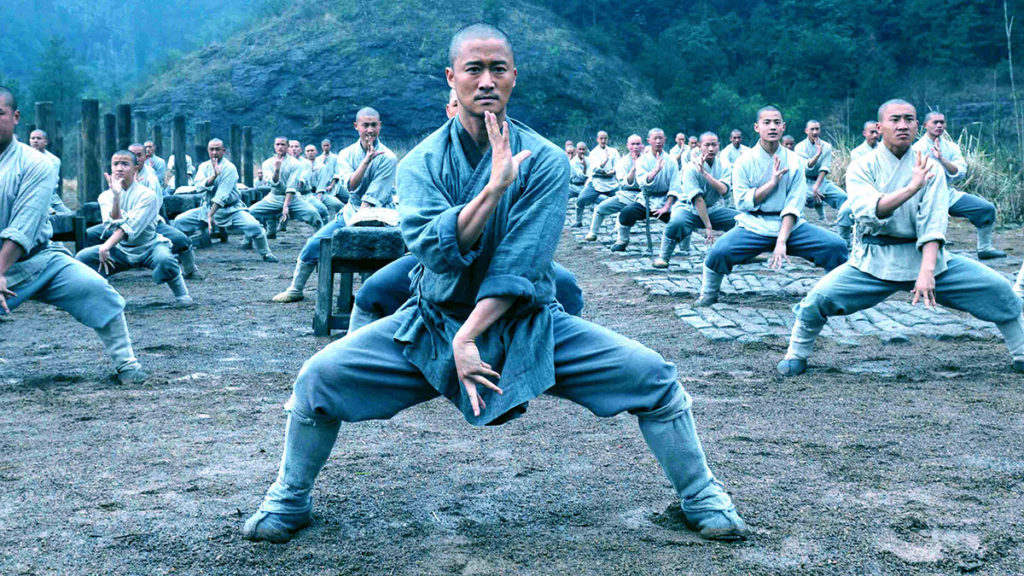This full-color outdoor image, possibly a screenshot from a movie, captures a group of Asian men practicing a martial art on a dirt field surrounded by green trees and hills. The men, all with shaved heads, are aligned in multiple lines, executing the same pose with meticulous precision. Each man has his legs extended in a crouch, facing forward, with his right arm held up in front of his face and his left arm positioned in front of his groin, fingers splayed.

The man in the forefront, presumably the instructor, stands out with a blue top contrasting the white tops worn by the others. He wears what appears to be a greenish robe-like garment, matching pants, and possibly high socks or soft shoes. His intense gaze is directed straight ahead, embodying focus and discipline. Some men have mats underneath them, but not all. The image evokes a sense of unity and synchronization amidst a serene natural backdrop.